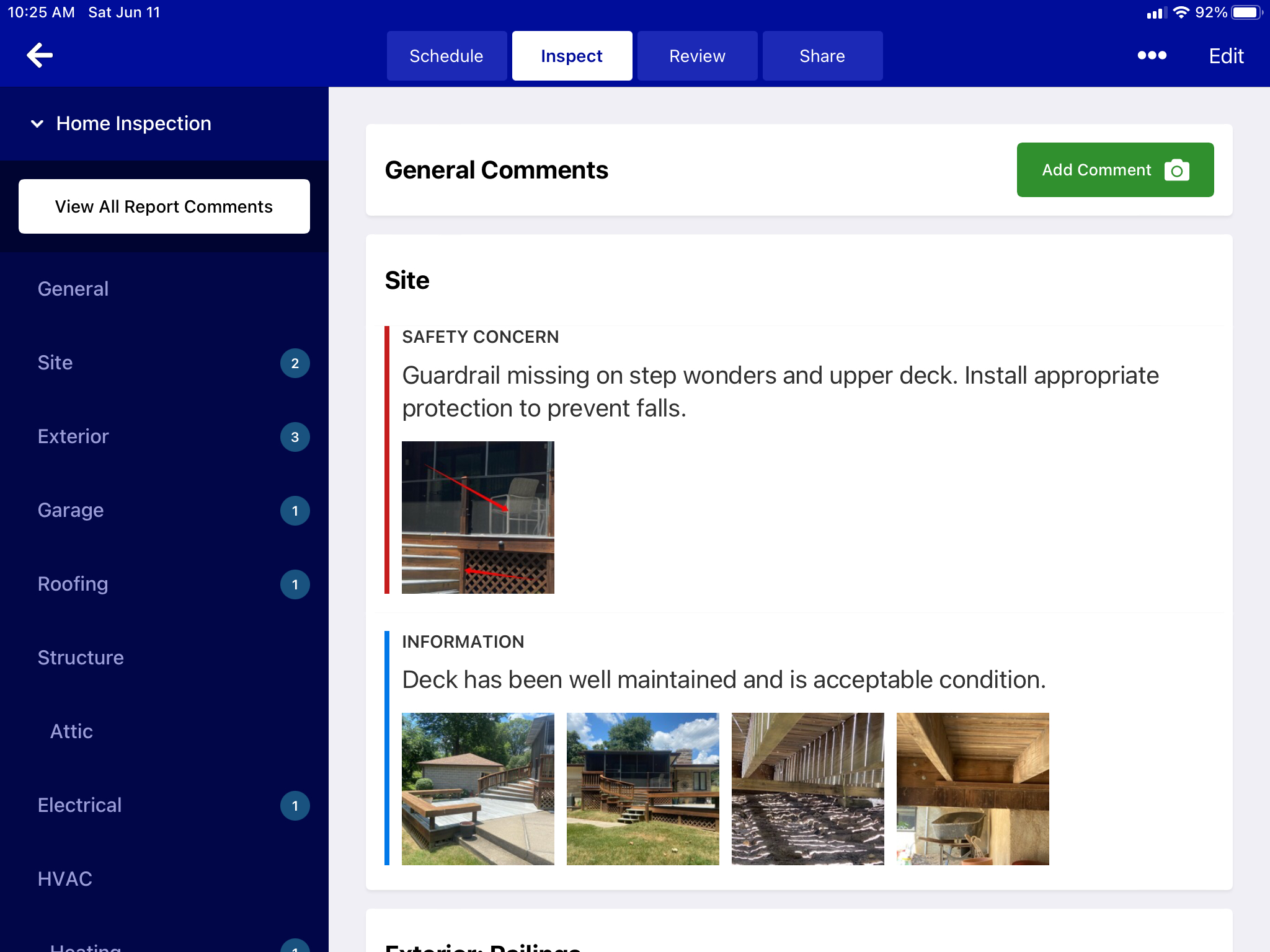**Caption:**

The image captures a screenshot of a home inspection app interface. At the top left, there is a blue header displaying "10:25 AM, Saturday, June 11." The header also features various options like "Schedule," "Inspect," "Review," and "Share," with "Inspect" being selected, indicated by a white rectangle with blue text, whereas the others are blue with white text. The battery level is shown as 92%.

Beneath the header, there are images depicting a site safety concern. One image highlights a missing guardrail on the steps and upper deck, along with a note suggesting the installation of necessary protection to prevent falls. Another note states that the deck has been well-maintained and deemed acceptable.

On the left side of the screen, there's a detailed navigation menu listing various inspection categories such as "Home Inspection," "View All," "Report," "Comments," "General," "Site" (with a number 2 beside it), "Exterior" (with the number 3), "Garage" (number 1), "Roofing" (number 1), "Structure," "Attic," "Electrical" (number 1), "HVAC," and partially cut-off "Heating" likely indicating number 1 as well.